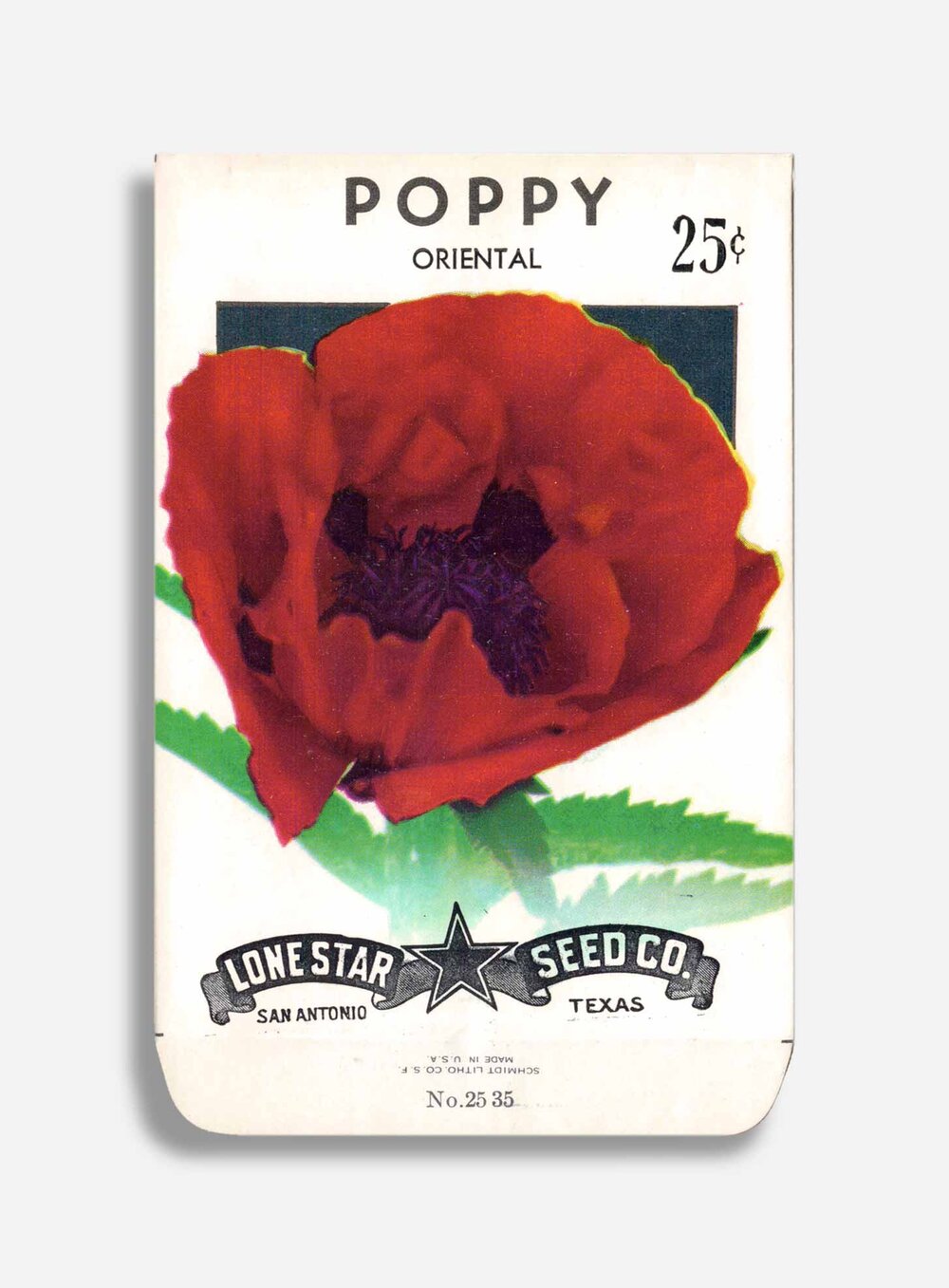This is a detailed illustration of a vintage seed packet set against a light gray background. The cream-colored packet features a vibrant, open red poppy with a black center, flanked by green leaves. At the top of the packet, in bold black text, it reads "Poppy Oriental, 25 cents." Below the poppy, a prominent black banner stretches across the bottom, with "Lone Star Seed Co" printed in white. A large star separates the text, with "San Antonio" written under "Lone Star" on the left and "Texas" under "Seed Co" on the right. The edges of the packet show signs of discoloration, reinforcing its vintage appearance. Additionally, the bottom flap bears the text "Number 2535," and an upside-down print above it reads "Schmidt Litho Company SF, made in the USA."